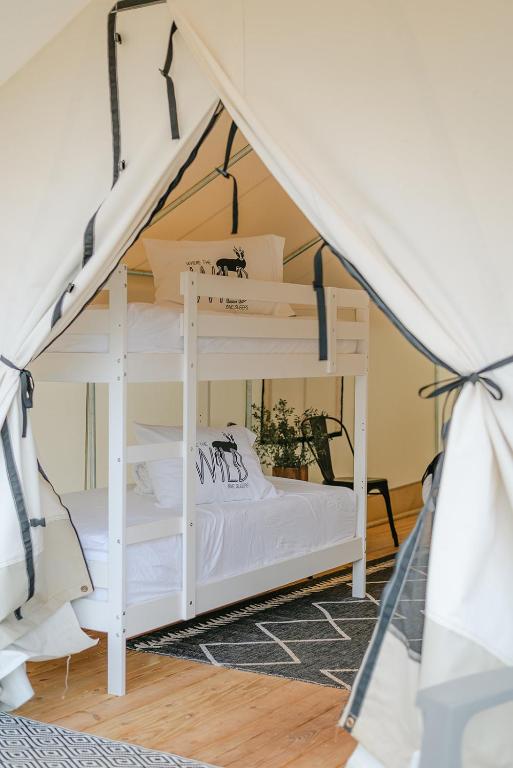The image depicts the interior of an elegant yurt-like tent, possibly situated indoors given the light brown hardwood floors. At the entrance, gray fabric curtains tied with matching ribbons create a welcoming doorway. Inside, the yurt is tastefully decorated with pure white bunk beds adorned with luxury throw pillows, including some featuring a black and white deer design with the word "wild". The floor is covered in two distinct rugs—a braided one at the entrance and a larger one in the center, both showcasing intricate diamond patterns in shades of gray and white. A green plant in a brown pot adds a touch of nature, positioned next to a sleek black chair. The overall ambiance is serene and sophisticated, blending rustic charm with refined decor.